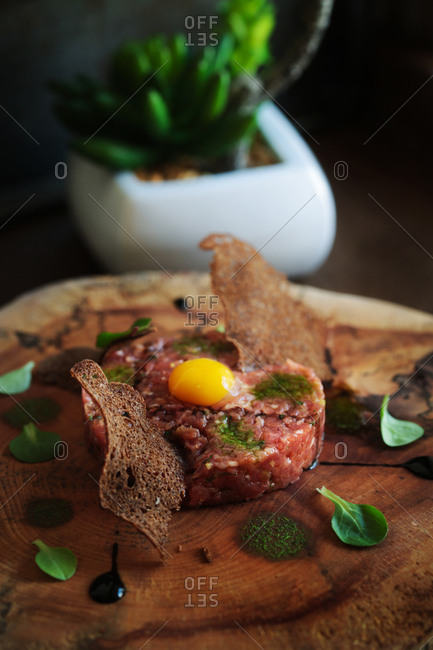The image showcases a meticulously arranged dish of tartare, which consists of a raw, circular meat patty, possibly made of ground beef or ground turkey. Centered atop the patty is a small, uncooked quail egg, its yellow yolk contrasting vividly with the meat. The patty is garnished with leafy greens and a drizzle of vinaigrette, adding a vibrant touch to the presentation. Two thin, toasted bread slices are artfully positioned to give the appearance of wings extending from the sides of the patty. The dish is presented on a rustic wooden serving plate, resembling a halved tree trunk, enhancing the natural aesthetic of the arrangement. In the blurred background, a vibrant green plant sits in a square white planter, adding a splash of color to the predominantly dark setting. Notably, the image features watermarks with the word "offset," subtly marking the visual.